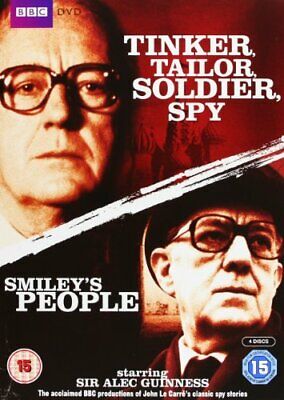The image is a detailed cover showcasing a BBC DVD release of two classic spy films, "Tinker Tailor Soldier Spy" and "Smiley's People", based on John le Carré's novels. In the upper left corner, there is the BBC DVD logo on a violet background. The composition features a diagonal split, separating two images of Sir Alec Guinness. On the top left, an older white man with short brown hair and round black glasses stares sternly at the camera against a red background, identified by the white text "Tinker Tailor Soldier Spy" above him. Below, the same man wears a round black hat, a black coat, a black tie, a white collared shirt, and the same black glasses against a black background, with the white text "Smiley's People" to the left. The bottom part of the image highlights in white text, "starring Sir Alec Guinness", emphasizing the acclaimed BBC productions of these iconic spy stories.